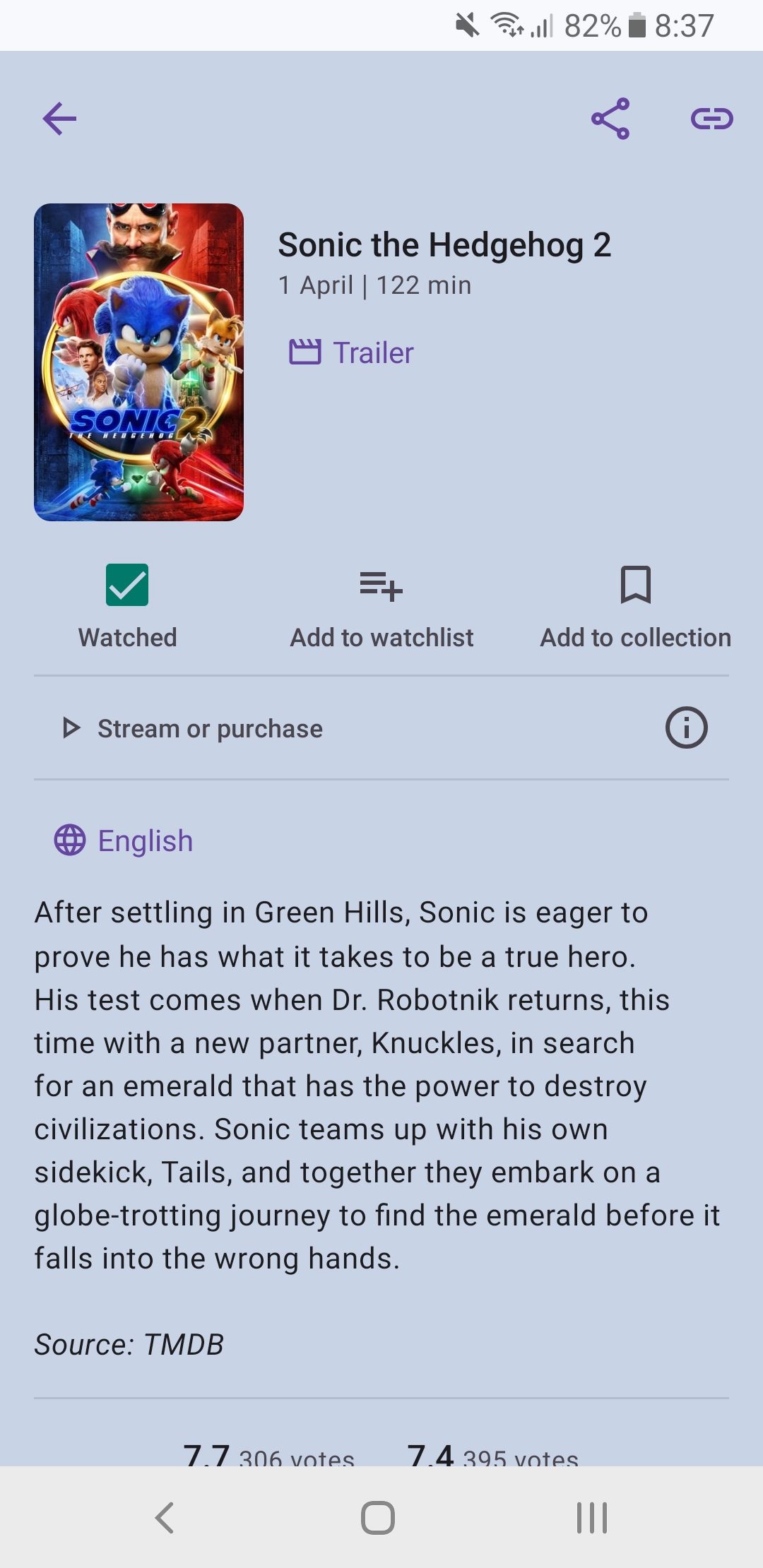This screenshot captures a user interface from what appears to be a movie streaming service, showcasing the film "Sonic the Hedgehog 2." The screen layout indicates it belongs to an app or service similar to Netflix.

At the top, the device's status bar is visible, showing the audio is muted, Wi-Fi signal strength at three out of four bars, battery level at 82%, and the time is 8:32. Below this, the interface features navigation elements including a back button, share option, and links positioned above the movie information.

In the forefront, there is a prominent thumbnail resembling a movie poster or DVD cover for "Sonic the Hedgehog 2." The background is a subtle washed-out blue, giving it a cohesive appearance. The poster features the villain in the backdrop, with Sonic the Hedgehog and an iconographic element prominently displayed.

Detailed movie information is provided just beneath the title, "Sonic the Hedgehog 2." The release date is marked as 1st of April, the runtime is listed as 122 minutes, and there's a purple button with a director’s clapboard icon labeled "Trailer."

Below this, three interactive options are shown: 
- A green box with a check mark labeled "Watched."
- "Add to watchlist" option.
- "Add to collection" option. 

Following these, there’s an option to either stream or purchase the movie. Additionally, a note reads "Purple Globe," indicating availability in English. 

The movie synopsis lays out the plot: After settling in Green Hill, Sonic aims to prove his heroism. His opportunity arises when Dr. Robotnik returns with a new accomplice, Knuckles, seeking an emerald capable of destroying civilizations. Sonic, along with his sidekick Tails, embarks on a global quest to prevent the emerald from falling into the wrong hands.

Lastly, the ratings provided show a 7.7 score based on 306 votes, and another 7.4 score from 395 votes, though the sources for these ratings are truncated and not visible.